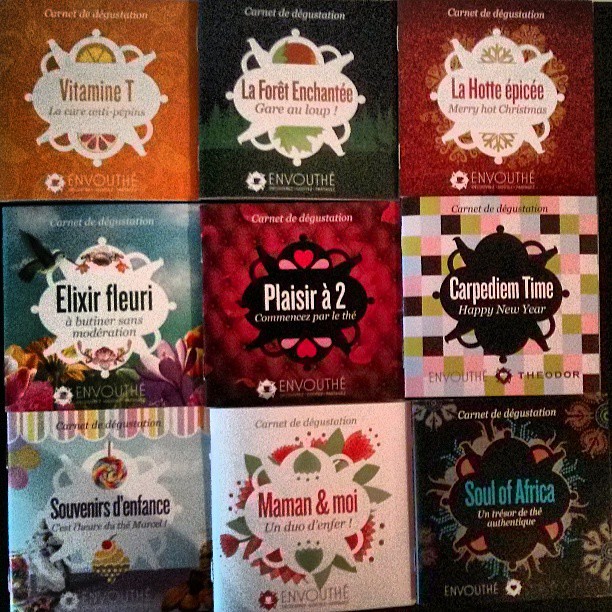The image depicts nine square publications, all sharing the same shape and format but with unique and colorful covers. Each cover prominently features a logo resembling two teapots stacked on top of each other, with French text in the middle. The top row, from left to right, includes: 

1. An orange publication labeled "Vitamine Tea" with citrus fruit imagery.
2. A dark green publication titled "Laforet Enchantée" with a forest backdrop.
3. A red publication called "La Hotte Epicée."

The middle row, from left to right, features:

4. A blue publication named "Elixir Fleurie," adorned with flowers and a bird.
5. A red publication "Plaisir A2" with heart motifs.
6. A multicolored, checkered publication stating "Carpe Diem Time, Happy New Year."

In the bottom row, from left to right, you find:

7. A publication with an ice cream and candy-themed cover titled "Souvenirs d'Enfance."
8. A white publication "Maman & Moi" decorated with red flowers.
9. A black publication "Soul of Africa" featuring nature-like patterns.